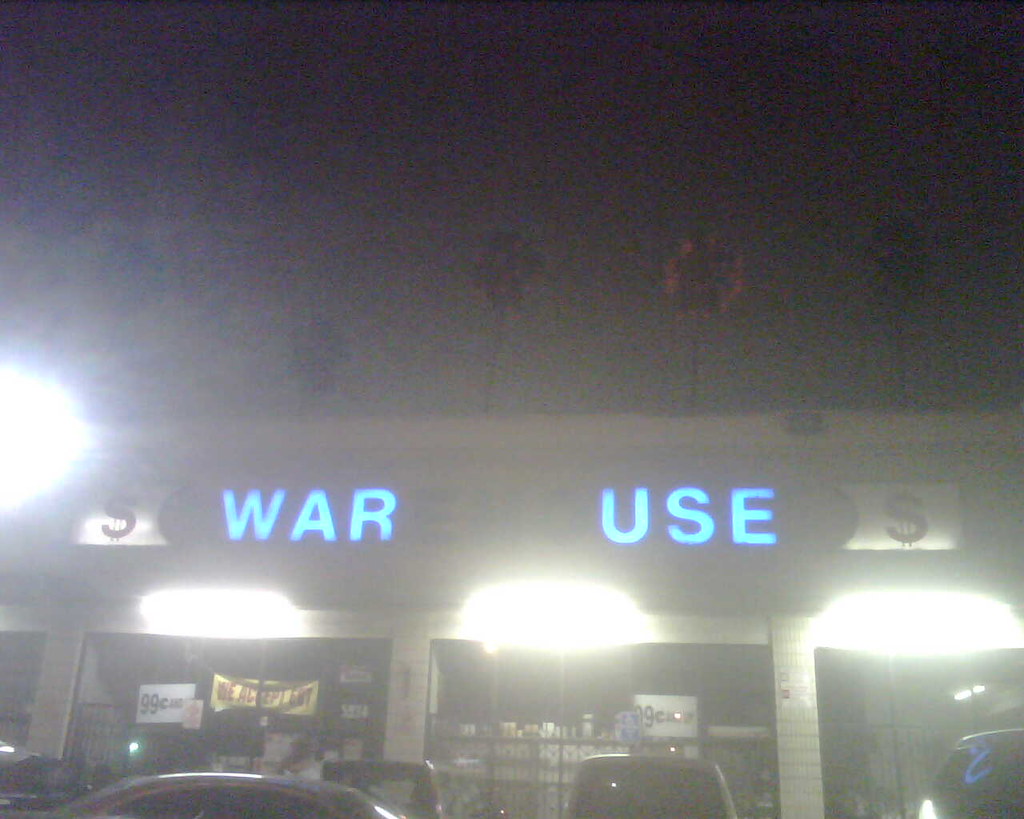Nighttime photograph of the front of a seemingly closed business establishment. The dark interior is visible through multiple windows, each showcasing merchandise with no illumination from within. Outside, the building is lit by bright lights framing the windows, highlighting a sign that reads "Warehouse," although the middle three letters are blacked out, leaving the illuminated blue letters to spell "War" and "Use." Additionally, there are dollar signs flanking these words. In front of the store, several cars are parked, and the window displays a yellow sign stating, "We accept EBT," as well as a white sign with bold black text advertising "99 cents."